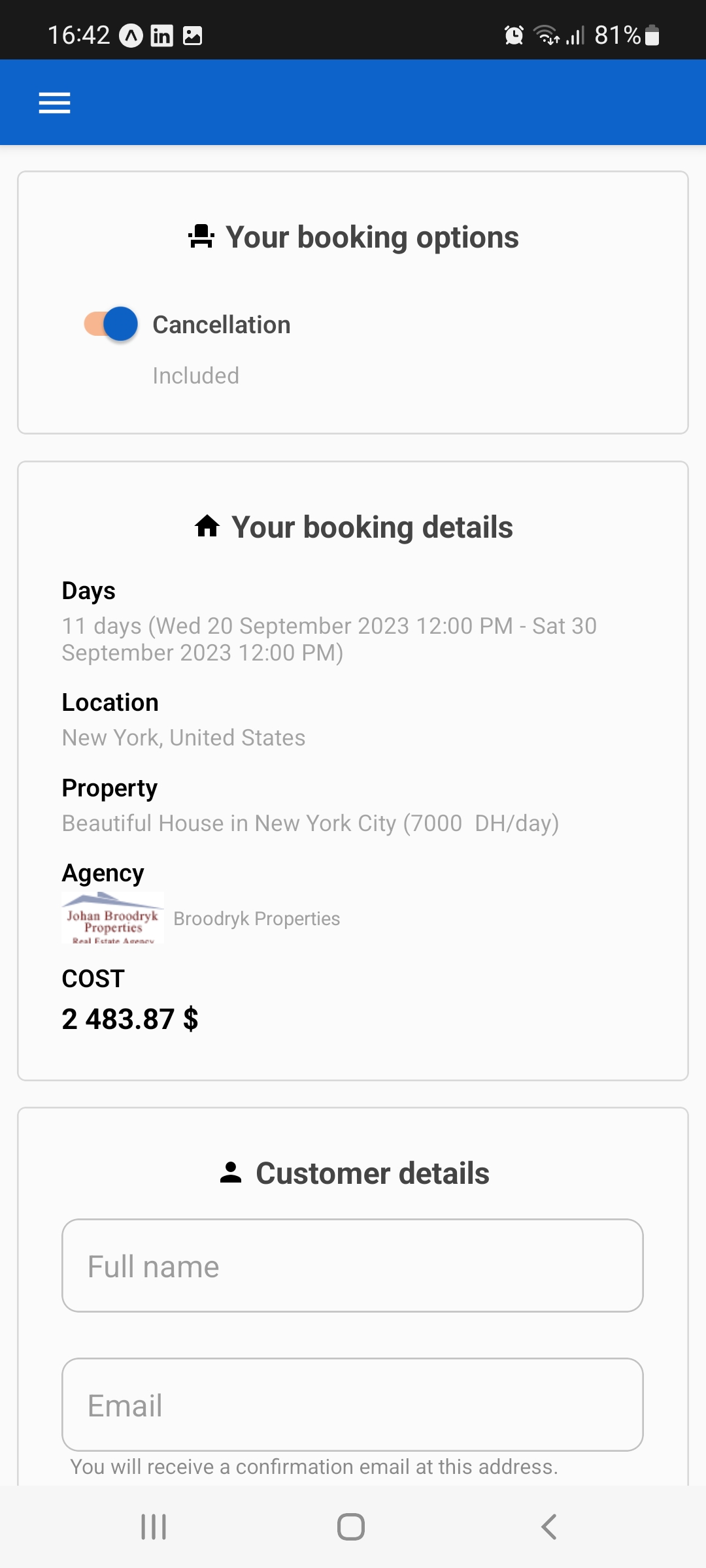At the top of the image, a long black bar displays the time as 16:42 on the left and the battery level at 81% on the right. Directly beneath this bar, there is a long blue bar with three tiny white horizontal lines on the left side. Below this blue bar, the text reads "Your Booking Options." Adjacent to this, it says "Cancellation," next to a blue circle partially filled with pink on the left.

Further down, under the section labeled "Your Booking Details," the caption states "11 days (Wednesday 20th September 2023, 12pm - Saturday 30th September 2023, 12pm)." Following this, the location is identified as "New York, United States" in black text. The next line in black text reads "Property: Beautiful house in New York City." The section labeled "Agency" is followed by the cost "$2483.87" with a black dollar sign next to it.

Below the cost details, the section "Customer Details" is presented with two open rectangles: one containing the placeholder text "Full Name" and the other "Email." At the very bottom center of the image, there is a small square icon.